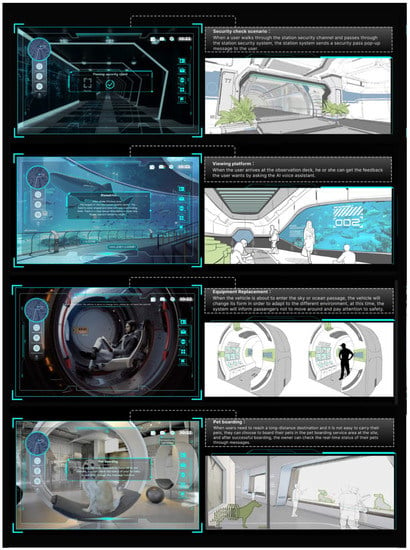The image is an 8-part series laid out in two columns and four rows, each contained within a vertical black frame. The left column features more realistic digital illustrations, while the right column showcases sketched versions of similar scenes. 

1. At the top left, there's a high-tech, black hallway with radar-type lines, evoking a futuristic or spaceship-like setting. Adjacent to it, on the right, is a grayscale sketch of a similar hallway structure.

2. The second image down on the left depicts an underwater scene with a large whale, resembling an advanced aquarium. To its right, a sketch portrays an aquarium with people standing in front of the glass, observing the marine life.

3. The third image on the left shows a circular pod interior with a person seated comfortably in a high-tech chair, suggesting a control room. The corresponding sketch on the right illustrates two pods with a standing figure rendered in shadow, emphasizing a more conceptual design.

4. The fourth and final image on the left displays a white dog sitting on a blanket within an open, circular seat, suggesting a cozy, enclosed space. In contrast, the sketch on the bottom right highlights dogs interacting with caregivers, emphasizing a more hands-on, nurturing environment.

This collection possibly serves as a comparison of detailed, realistic renderings against their conceptual, sketched counterparts, potentially from a training manual or instructional guide.